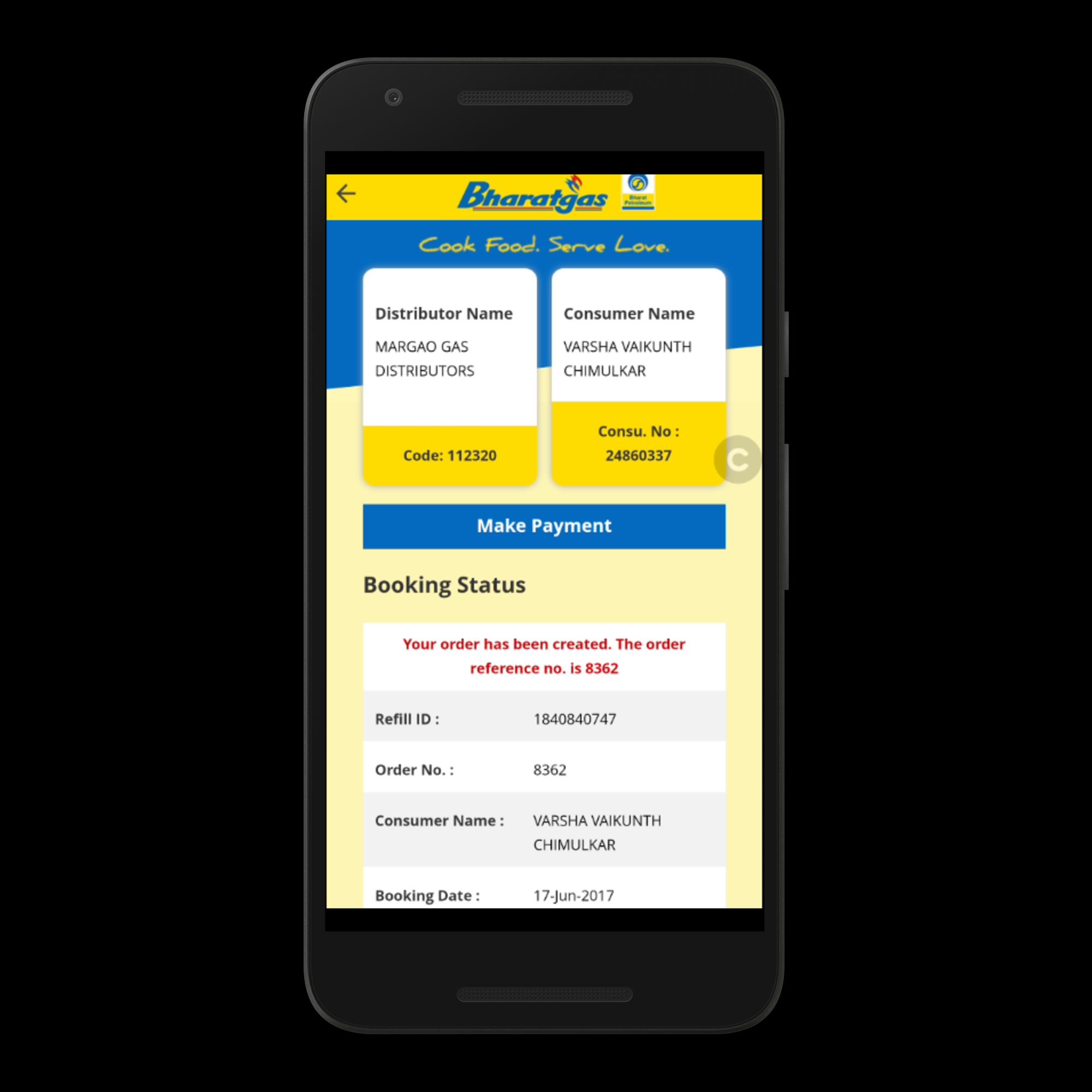This image is a top-down photograph of a black smartphone against a solid black background. The screen is displayed clearly, though there is a slight clipping where the phone’s frame is distinguishable from the main display.

At the top of the screen, there is a horizontal yellow bar. Directly below this bar is the name "Barrett Gaske" in blue text with a red underline. Beneath this name, there is a slogan, "Cook Foods Serve Love," rendered in yellow italics.

The upper section of the screen features a blue background. At the bottom of this section, "Distributor Name: Margaret Barrett Gaske" is written, with "Distributor" positioned to the right. Next to it is "Consumer Name: Barska Van Cleef, Schumacher."

Below these details, there is a space for a code that appears to track the consumer on the right. The phrase "Make Payment Below" is prominently displayed, followed by "Booking Status." In red text below, it states, "Your order has been created. The order reference number is 8362." The number "8362" is repeated in the context of "Order Number," with an additional "Refill ID: 1-8-4-8-4-0-7-4-7."

Further down the screen, it reiterates "Order Number: 8362" and "Consumer Name" once again. Finally, it finishes with "Booking Date: 17 June 2017," with the date separated by dashes.